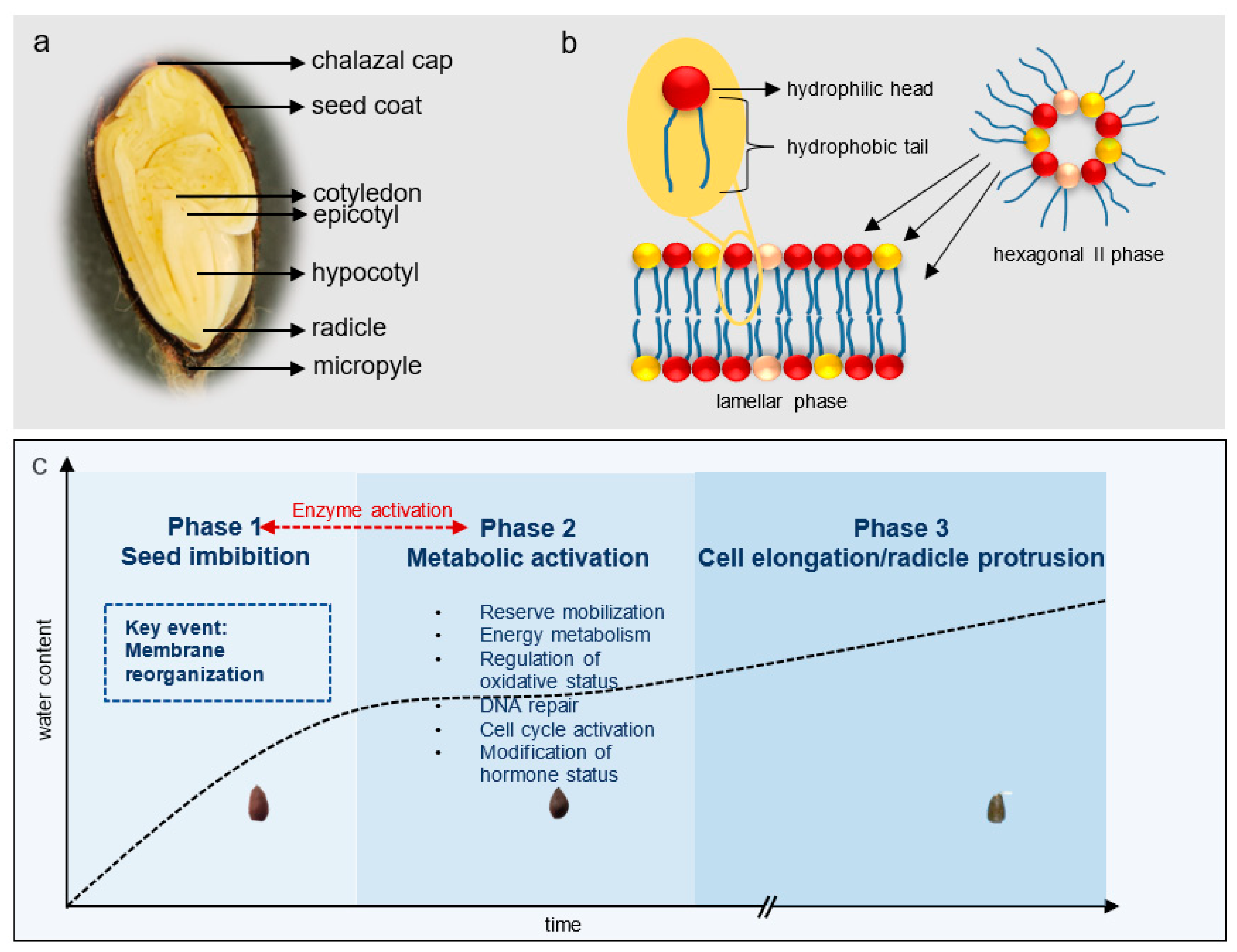This detailed diagram is an instructional and educational image on seed anatomy and growth phases. The horizontal rectangular image is divided into two main sections, with a light purple background on top and a white background on the bottom. The upper section is further divided into two labeled parts, 'A' and 'B'.

In part 'A' on the left side, there is a diagram of a seed cut in half, with black arrows pointing out and labeling various parts such as the seed coat, shizzle cap, cotyledon, epicotyl, hypocotyl, radicle, and micropyle. These labels indicate the internal and external components of the seed, providing a detailed view of seed anatomy.

Part 'B', located at the top right, contains colorful images that look like molecular structures. There is a yellow oval with a red circle and blue lines, with black arrows indicating parts such as the hyphrololic head and hyphropybolic tail. Additionally, there are mirrored yellow and red dots with a pearl-colored center and blue strings, labeled as the lamir phase. The diagram also shows the hexagonal 2 phase, represented by a circular arrangement of yellow, red, and pearl-colored circles with tails facing outward.

The bottom section, labeled 'C', features a blue graph on a white background, depicting the water content over time through different phases of seed growth. The graph has an upward diagonal line intersecting three distinct phases. Phase 1, in light blue, covers seed inhibition and key events like membrane reorganization and enzyme activation. Phase 2, in darker blue, encompasses metabolic activation with details on reserve mobilization, energy metabolism, regulation of oxidative status, DNA repair, cell cycle activation, and hormone status modification. Phase 3, in the darkest blue, includes cell elongation and radicle protrusion. The graph's dotted line highlights the increasing water content from phase 1 to phase 3.

Overall, the image is a comprehensive and color-coded visual guide to the anatomy of a seed and the stages of its growth, aimed at providing detailed scientific information.